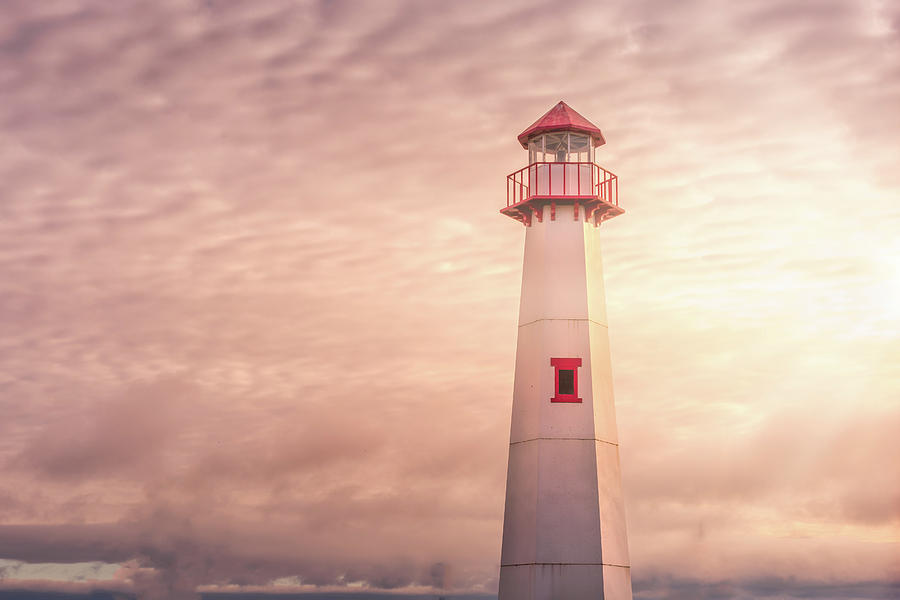The image features a tall, predominantly white lighthouse set against an incredibly cloudy sky illuminated by sunlight breaking through from the middle right-hand side. The sun's rays cast a warm palette ranging from red-orange to white-yellow over the clouds. The photograph is taken from the ground, looking up at the lighthouse, which is positioned slightly off-center to the right. The lighthouse itself has four visible sections with distinctive red detailing: a red peaked roof at the top, a catwalk with red railings encircling it just below, and a single window outlined in red located on the second section from the top. The lighthouse has a textured appearance, with some areas suspiciously white, lending it an almost video-game-like quality. The detailed red and white elements, along with the intricate sky, combine to create a striking and ethereal scene.